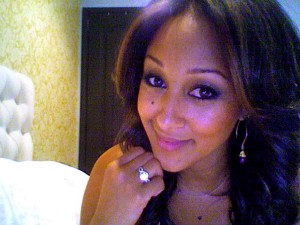In the image, a woman who slightly resembles Tiffany Haddish is captured in a close-up shot, resting her chin on the knuckle of her left hand, which is adorned with a silver ring. She has big eyes, pencil-thin black eyebrows, and red lips. A notable beauty mark is present under her left eye. Her dark, flowy hair frames her face, and she sports two dangly earrings and a necklace with a black stone. The background features a white bed with a soft headboard to the left, a white pillow, a yellow wall with floral wallpaper, and a dark brown door. The woman is staring directly at the camera, smiling gently.